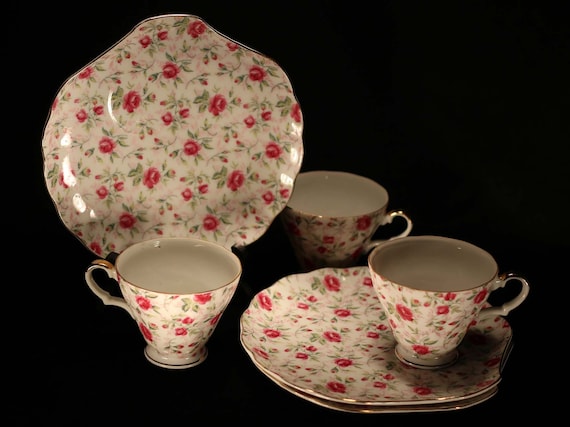This photograph showcases an elegant set of china dinnerware against a stark black background. The set features a distinct red floral design with green leaves and stems, which gracefully decorates each piece in a slightly varied, yet harmonious, pattern. Central to the image is an upright plate, adorned with red flowers in various stages of bloom, from buds to fully open blossoms. Positioned below this standing plate is a teacup bearing the same intricate floral motif. To the right, another teacup stands alone, mirroring the design. Additionally, two plates are neatly stacked at the bottom right, with a third teacup placed atop them. The entire surface of each plate and cup is embellished with the red flowers and green foliage, creating a cohesive and charming aesthetic throughout the set.